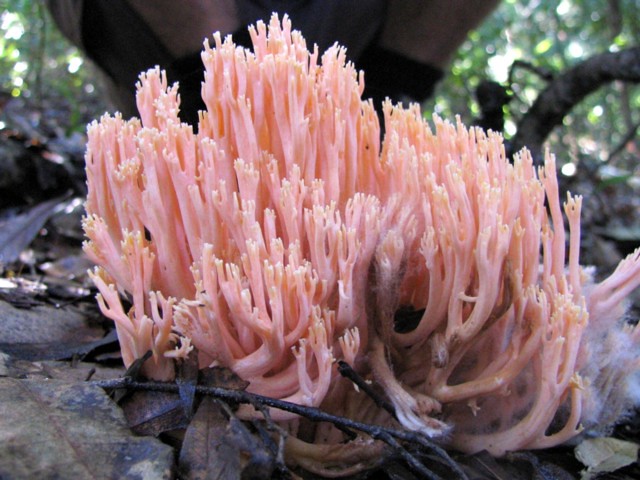The image is a detailed, professionally-taken photograph of a unique cluster of fungi in a forest setting. The fungi, which appear pink with delicate, flesh-colored tubes, are growing vertically from the ground, surrounded by dark brown leaves and foliage. At the ends of these tubes are small nubs or, as some might interpret, yellow-tipped tiny hairs, but they lack traditional mushroom caps. The background features nearly black-brown branches and green leaves, with sunlight softly filtering through, creating a beautiful depth of field that highlights the sharply focused fungi against a blurred woodland backdrop. The overall scene is reminiscent of coral or sea life due to the fungi's unusual appearance and coloration.